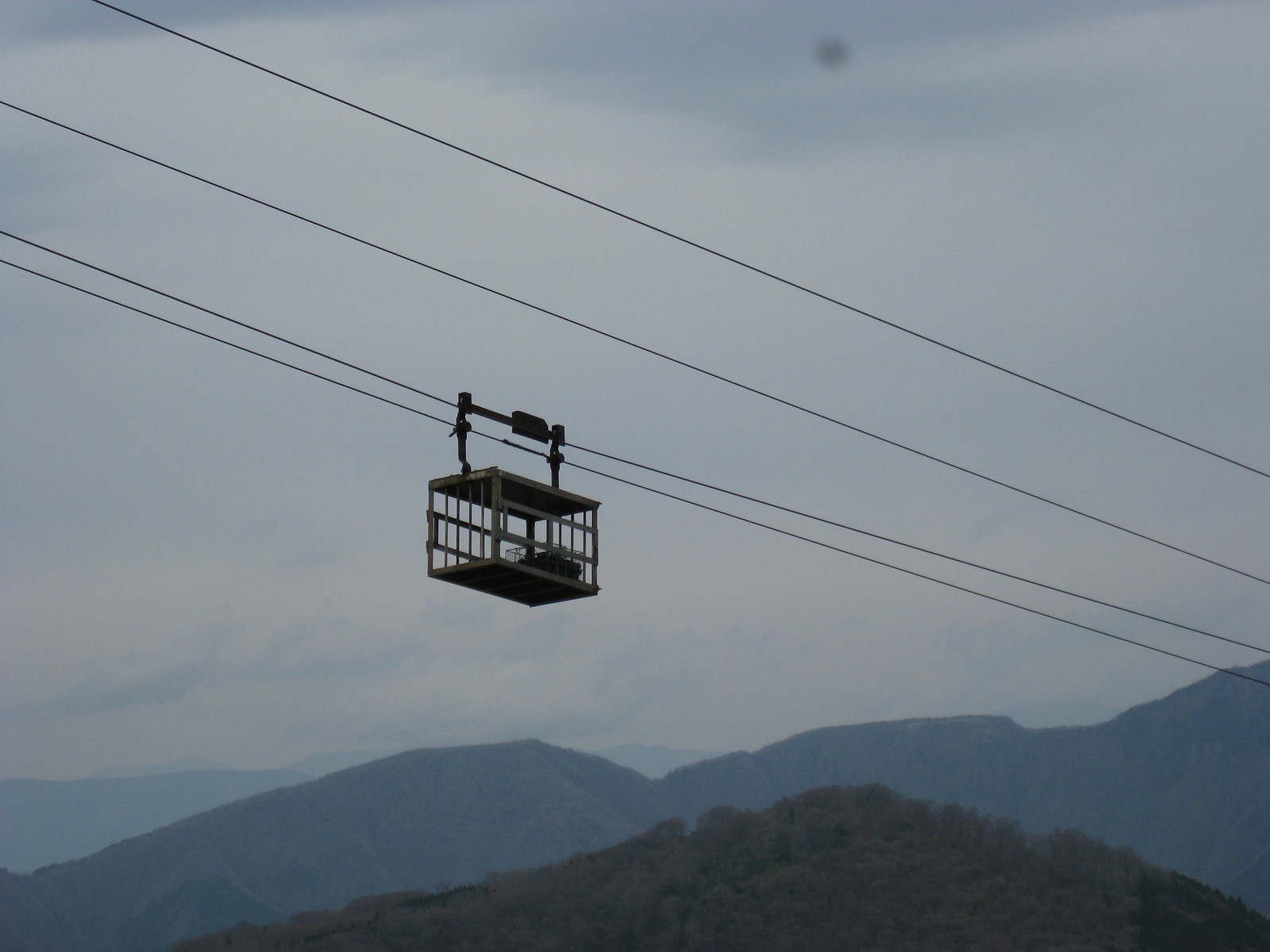The image captures an outdoor scene featuring a metal cage suspended high in the air via four wires that extend from the upper left corner diagonally down to the right. The cage, which is rectangular with a solid bottom and top, centers the frame, hanging from a horizontal arm attached to the cables above. This metallic structure has bars on all its sides, except for an open section on the back left. Below the cage, rolling green hills densely covered with vegetation dominate the foreground. Farther back, a taller, partly shadowed mountain rises, its terrain a blend of yellow and white. The overcast sky is filled with clouds that transition from white at the bottom to darker grays at the top, and there is a distinct dark gray spot near the center-top of the sky. The scene exudes a tranquil, possibly early morning or late evening ambiance, enhanced by the cloudy sky and the different hues of green, gray, blue, white, and brown.